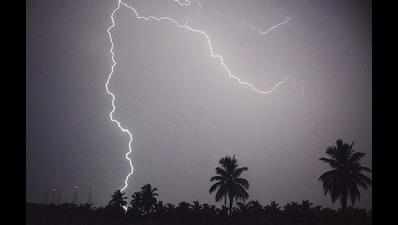The image is a dramatic black and white photograph that vividly captures a lightning strike. In the foreground, a series of dark silhouettes outline the scene, dominated by an assortment of palm trees. To the bottom right, two taller palms stand prominently in the center and mid-right, while three smaller palm trees form a group on the left side of the image. The horizon sits low at the base of the picture, creating an expansive view of the sky above. 

The sky itself is a heavy, imposing gray, providing a stark backdrop that fades out to black on either side. It's interrupted only by an electrifying display of lightning that splits the image. The main lightning bolt branches out from the upper center, forming two paths: one extends in a zigzag motion vertically down the left, reaching the bottom of the image, and the other stretches diagonally towards the right, forming an inverted V shape without the horizontal bar.

Additional bursts of light from three distinct bolts pierce through the dense sky, illuminating the otherwise dark and eerie scene. Subtle hints of buildings appear faintly at the distant left, adding an extra layer of depth to this somber, electrified landscape.